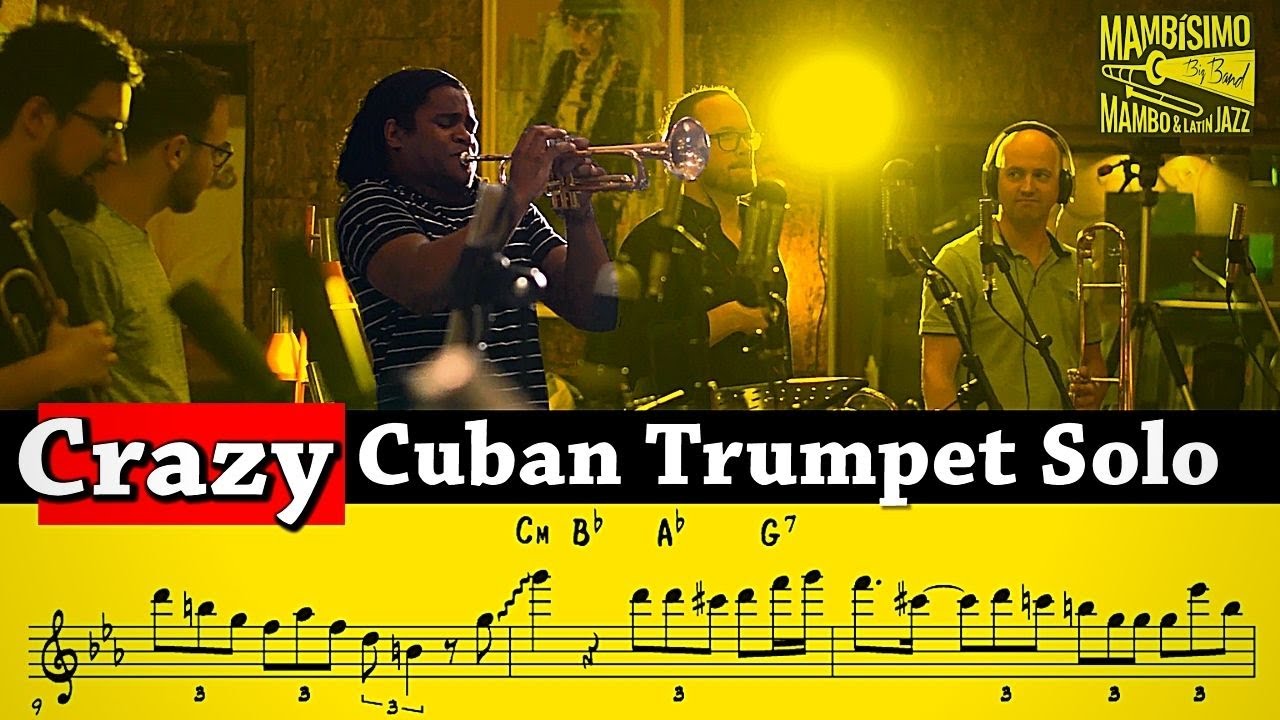This promotional image for Mambisimo, a Mambo and Latin Jazz Big Band, prominently features a studio recording session with five musicians. The upper right corner of the image shows the band's logo, "Mambisimo," spelled M-A-M-B-I-S-I-M-O, alongside a trumpet graphic. In the foreground, a darker-skinned man, possibly Cuban or African American, stands out as he passionately plays a trumpet, wearing a black-and-white striped shirt. The rest of the band members are somewhat obscured by a yellow haze but can still be identified; two light-complexioned men with glasses and beards are on the right, one holding a horn and the other in a light blue shirt without an instrument. Another man with scruffy hair and glasses stands to the left of the trumpet player, wearing a black shirt and holding an unidentified object. The final member, in a short-sleeved green shirt with headphones, holds a French horn and is looking at the other members. At the bottom of the image, a yellow rectangle displays musical notes on a scale labeled "9-3-3-3-3-3-3" and "C-M-B" with a higher "B," an "A" with a higher "B," and a "G7," accompanied by the text "Crazy Cuban Trumpet Solo," which is positioned in red and black rectangles with white lettering. The visual elements collectively emphasize the band's dynamic and vibrant musical atmosphere.